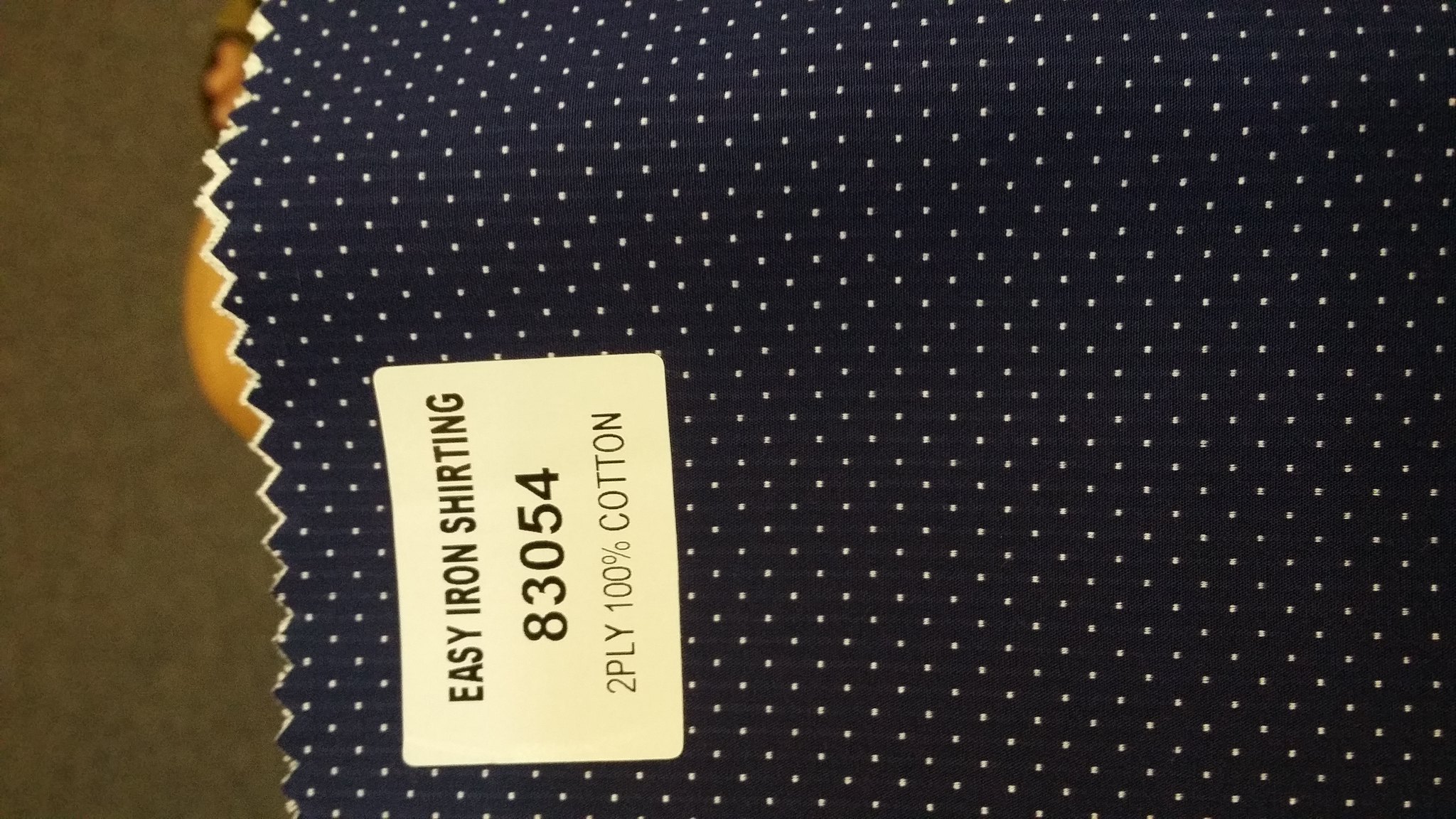This photograph features a sheet of midnight blue fabric adorned with a delicate pattern of small white dots. A small, white label is affixed to the left side, displaying the text "Easy Iron Shirting," along with the number "83054," and the material description "2 ply 100% cotton," all inscribed in black font. The fabric is draped over what appears to be a light wood stool or chair. The background comprises a medium gray floor or carpet, offering a subtle contrast that highlights the rich color and texture of the fabric.